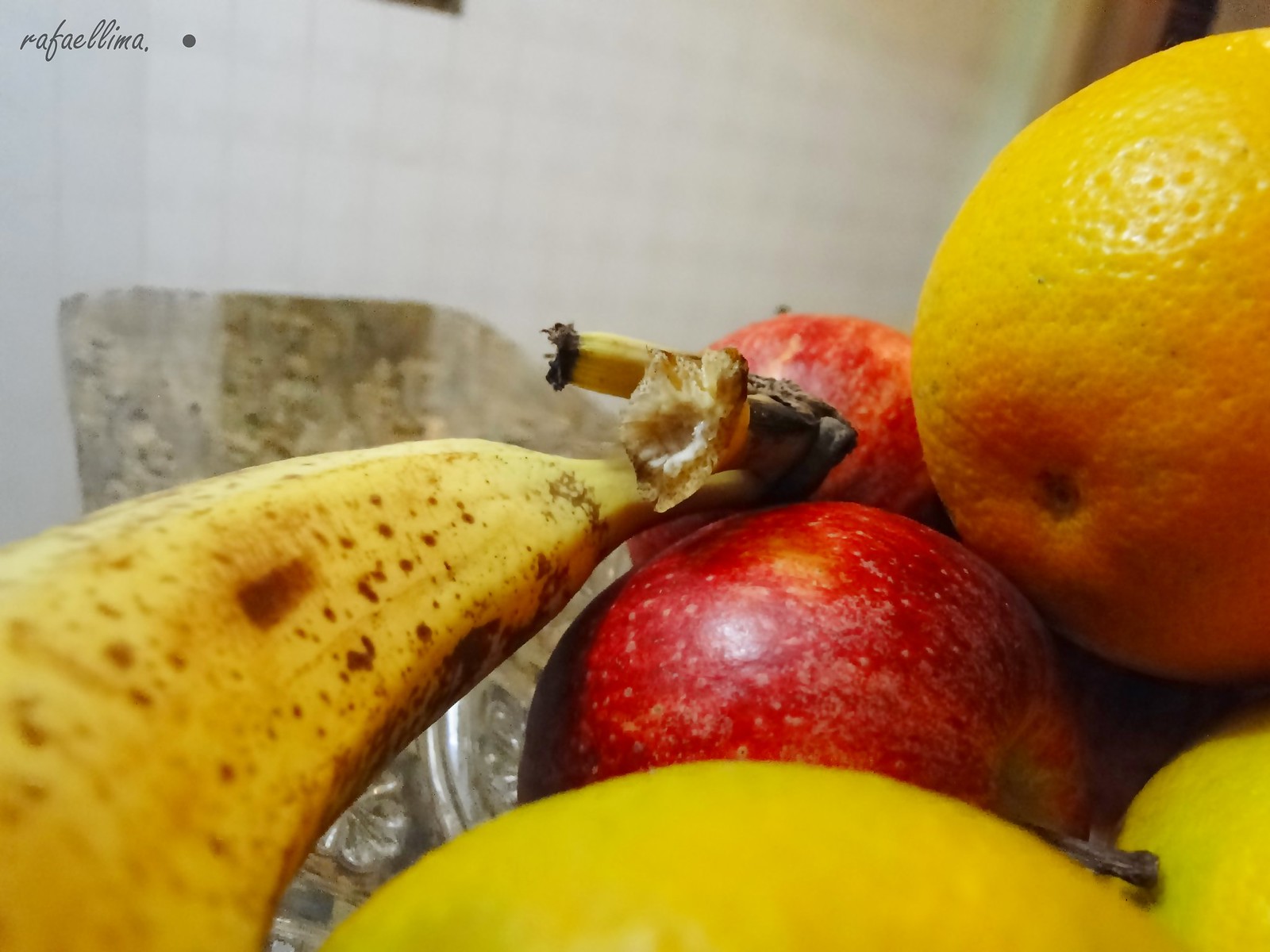Close-up of a fruit arrangement on a kitchen island. 

In the top left of the image, the word "RafaelLima" is elegantly written in cursive. The background features a kitchen wall adorned with small, white tiled squares. The narrow kitchen island beneath has a marble texture, blending light brown, dark brown, and black hues. Occupying the bottom right of the image, a bunch of fruits includes a yellow banana with a couple of broken stems, dotted with brown spots. Beside it, there is a red apple dusted with a bit of white, its stem still attached, with another apple partially visible behind it. An orange peeks out from the bottom of the arrangement, and two more oranges are slightly obscured beneath it. In total, six fruits make up this vibrant display.